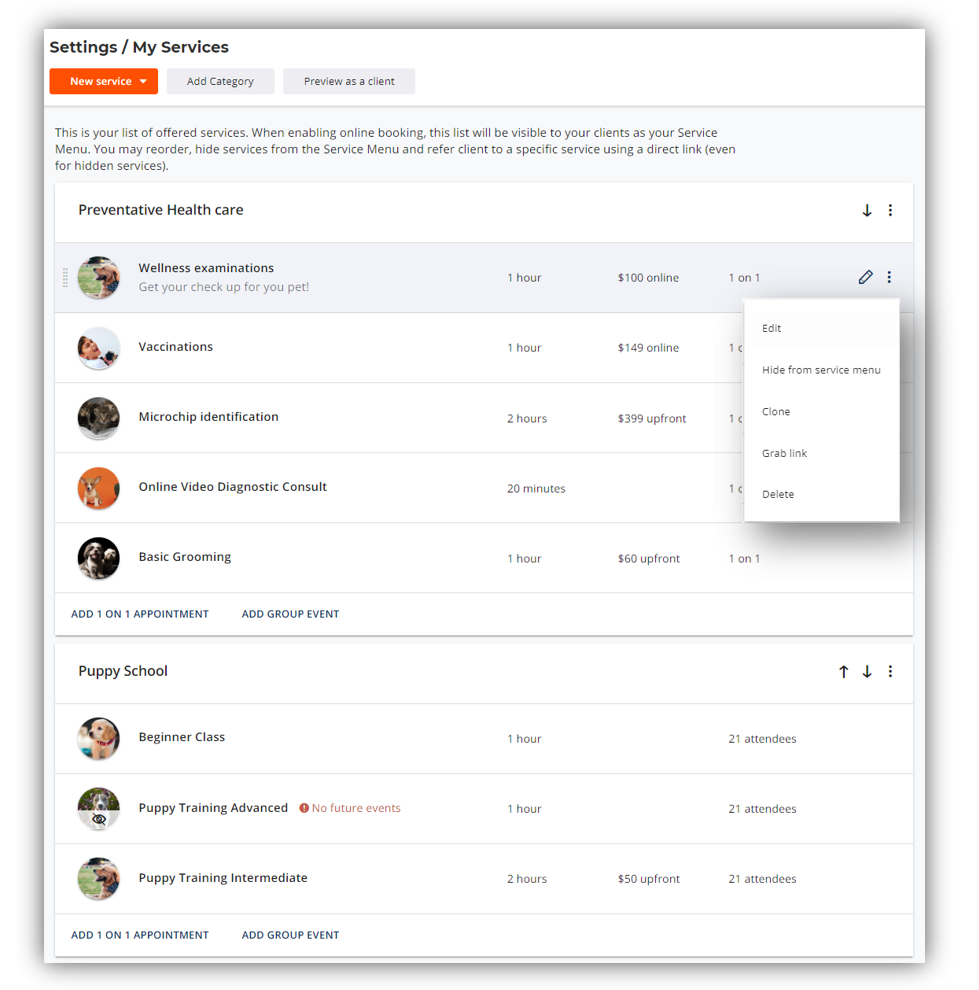This screenshot from a desktop application showcases the "Settings / My Services" section. At the top left, a prominent "New Service" drop-down button is highlighted in orange. To its right are two grayed-out buttons labeled "Add Category" and "Preview as a Client." Beneath this header, a grayish background displays an informational message: "This is your list of offered services. When enabling online booking, this list will be visible to your clients as your service menu. You may reorder, hide services from the service menu, and refer clients to a specific service using a direct link, even for hidden services."

The list begins with "Preventative Healthcare," which features a downward-pointing arrow and a vertical ellipsis (three dots) for additional settings. The first service listed under this category is "Wellness Examinations," highlighted in gray. Accompanying this entry is an image of a dog and a description: "Get your checkup for your pet. One hour, $100 online, one-on-one." An adjacent pencil icon offers options such as Edit, Hide from Service Menu, Clone, Grab Link, and Delete. To the right, the vertical ellipsis appears again for additional settings.

Following "Wellness Examinations," the list includes services titled "Vaccinations," "Microchip Identification," "Online Video Diagnostic Consult," and "Basic Grooming," providing a comprehensive overview of the service offerings.